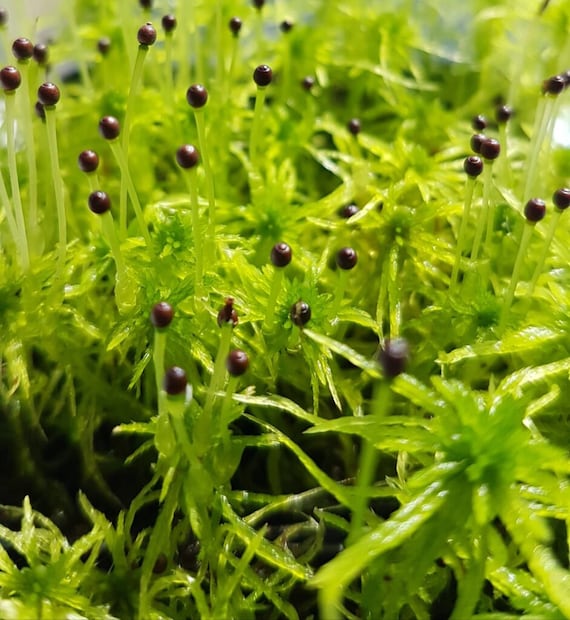This image is an extremely close-up, almost microscopic view of green plants, filling the entire frame with vivid detail. The photo is very bright and predominantly green, with thick, abundant grass and leaves taking up the majority of the scene. Emerging from the green plants are small, dark brown to black bulbs that resemble little antennas or round berries. These bulbous structures, roughly shaped like tiny olives, are numerous—potentially around 24 to 30 scattered throughout the image. The green stems and leaves appear slightly wet, adding a reflective sheen to the close-up shot. The background is blurred and somewhat dark, further accentuating the vibrant greenery and intricate details of the plant structures.